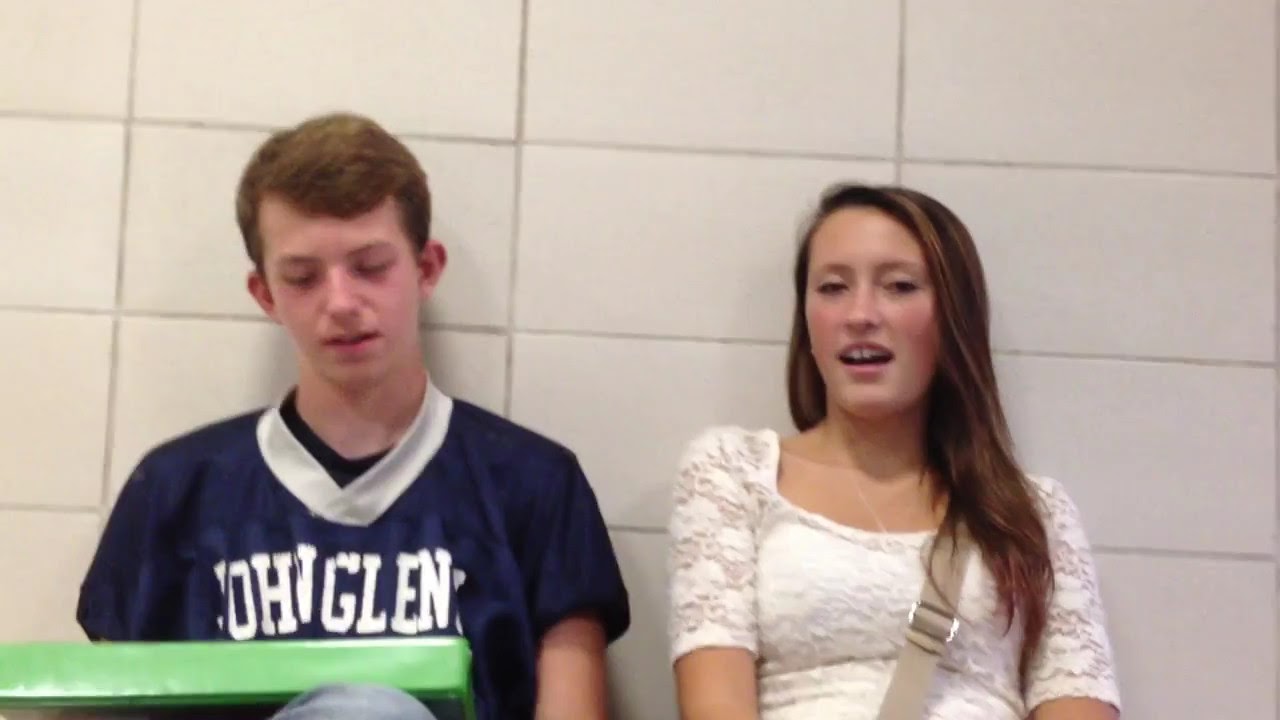The picture depicts an indoor scene with two Caucasian teenagers leaning against a white wall made of large tiled sections separated by grout. On the left is a young boy with short, reddish-brown hair feathered to the side, who has a red complexion. He is wearing a blue short-sleeved jersey with a white collar over a black shirt, and the writing on his jersey appears to say "John Glenn." The boy is sitting with his knees folded up and is looking down at a green board on his lap. To his right is a teenage girl with long, straight brown hair with streaks of blonde. She is wearing a white shirt that features lacy sleeves and has a beige strap, possibly for a purse, slung over her shoulder. The girl has a slightly red complexion and is looking toward the camera with her mouth open as if she’s talking.